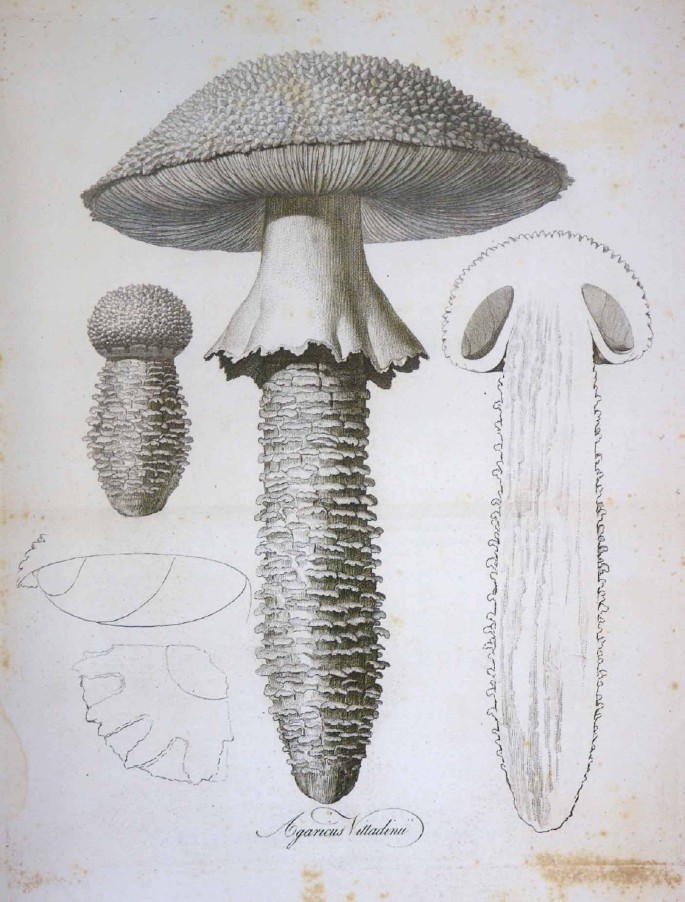This detailed botanical drawing showcases various views and stages of a single mushroom species, presumably created with pencil on white paper that has aged to a grayish tone, adorned with tan spots. Prominent cursive writing, likely the mushroom's scientific name, is delicately inscribed at the bottom, though it has become hard to decipher over time. The central focus of the illustration is a large, lifelike mushroom depicted with meticulous detail, emphasizing the stem and cap. To its right, an intricate cross-section reveals the mushroom’s internal structure, while to the left, a smaller, juvenile mushroom displays its nascent cap and root system. Faint pencil outlines in the lower left hint at an additional, possibly unfinished element. Throughout the drawing, a spiky texture on the cap contributes to a distinctive, lifelike appearance. The artist’s signature is subtly visible at the bottom, further authenticating this scientifically styled depiction.